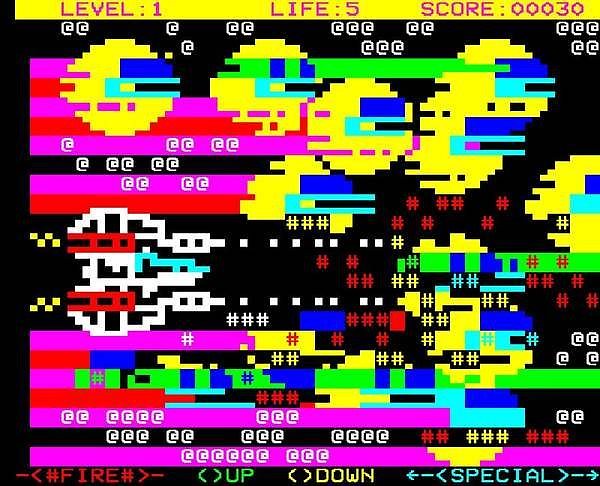The image is a chaotic and colorful screen capture resembling a glitched version of a classic video game, likely an old Atari game similar to Pac-Man. The screen is filled with a jumbled configuration of vibrant shapes and colors, including yellow dots, red stripes, purple, turquoise, black, white, and lime green. Yellow distorted circles dominate the top of the screen, with two white shooter elements in the center targeting degraded yellow circle objects. The background is black, creating a stark contrast with the bright, neon-like colors. Across the top, text indicates "Level 1," "Lives 5," and "Score 00030." Along the bottom, instructions read "Fire," "Up," "Down," and "Special." The image gives the impression of an old video game error screen, evoking nostalgia for classic games like Pac-Man and Frogger, with symbols and colors spiraling into visual chaos.